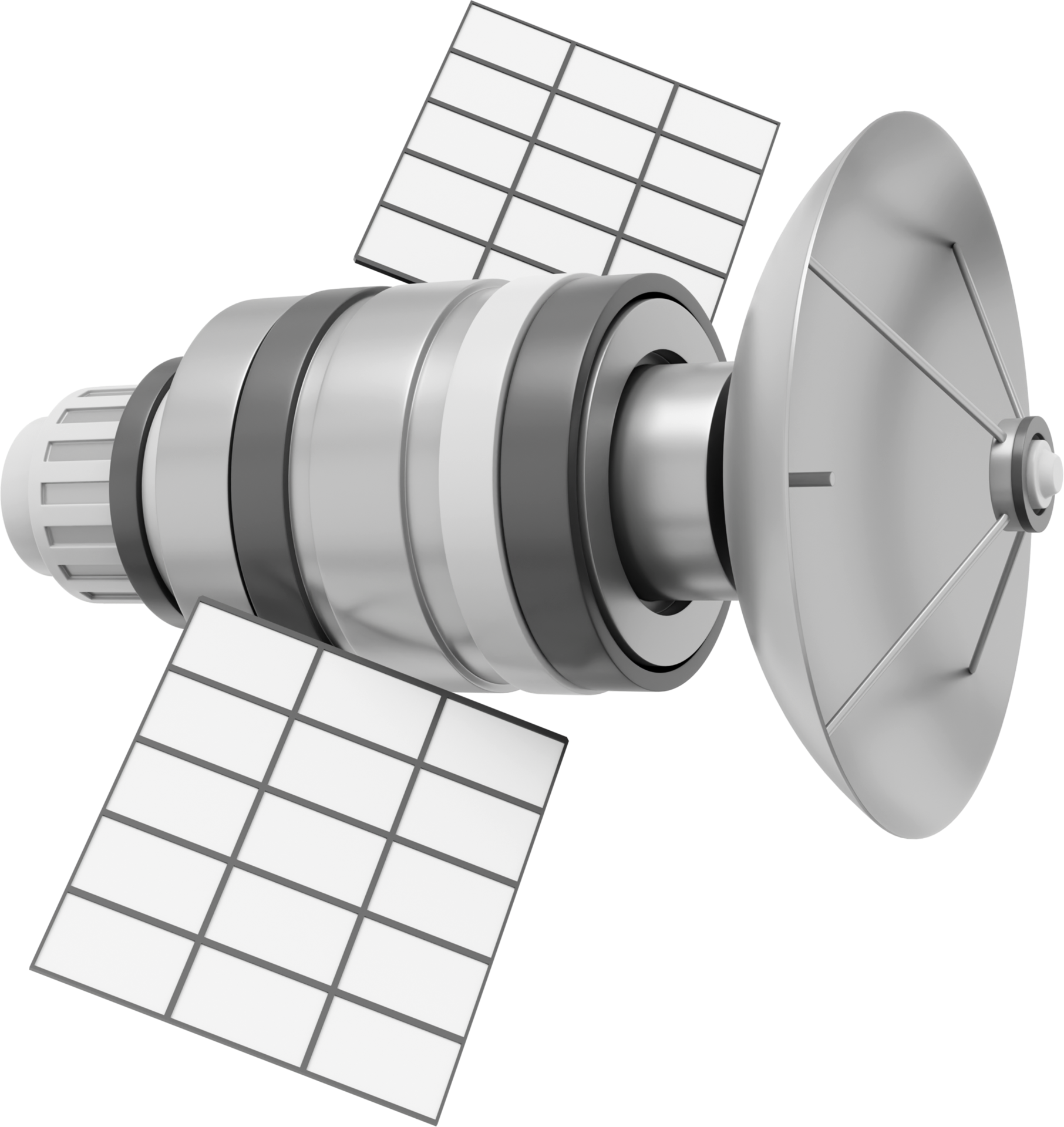The image depicts a highly detailed 3D illustration of a space satellite, predominantly in shades of gray and white. The satellite features a central cylindrical body composed of dark gray, light gray, and almost white bands, some of which include fluted indents. Extending from this central cylinder are two prominent rectangular solar panels, each divided into 15 segments arranged in a 5x3 grid with white centers and black borders. Additionally, on the far end of the satellite, there is a disc-shaped component, likely an antenna, boasting a four-pronged structure. The overall design is symmetrical, with the satellite positioned centrally in the image, highlighting its intricate metallic structure and diverse gray color palette.